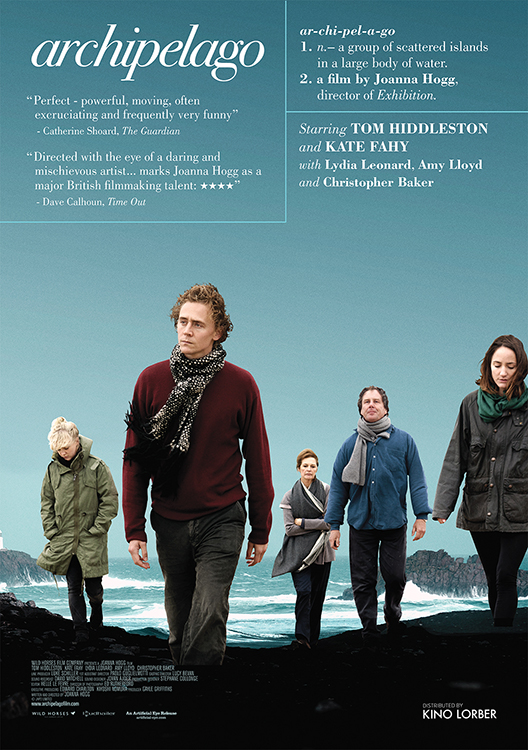This image is an advertisement for a movie titled "Archipelago." The background features a stormy sea with white foam on the waves, set against a bluish-gray sky. Prominent rocks jut out from the water on both the left and right sides. In the foreground, a dark, almost black rock shelf serves as a platform for five people, who are dressed in winter clothing, including jackets, pants, and some with scarves, suggesting a cold environment. The positioning of the people indicates they may have just emerged from the ocean. At the top of the image, in white letters, the title "Archipelago" is prominently displayed. Below the title, there are two quotes: one from Catherine Shore of The Guardian that reads, "Perfect, Powerful, Moving, Often Excruciatingly and Frequently Very Funny." To the right of the quote, "Archipelago" is defined in a two-point list. Lower down, text announces that the movie stars Tom Hiddleston and Kate Fay, alongside Lydia Leonard, Amy Lloyd, and Christopher Baker.